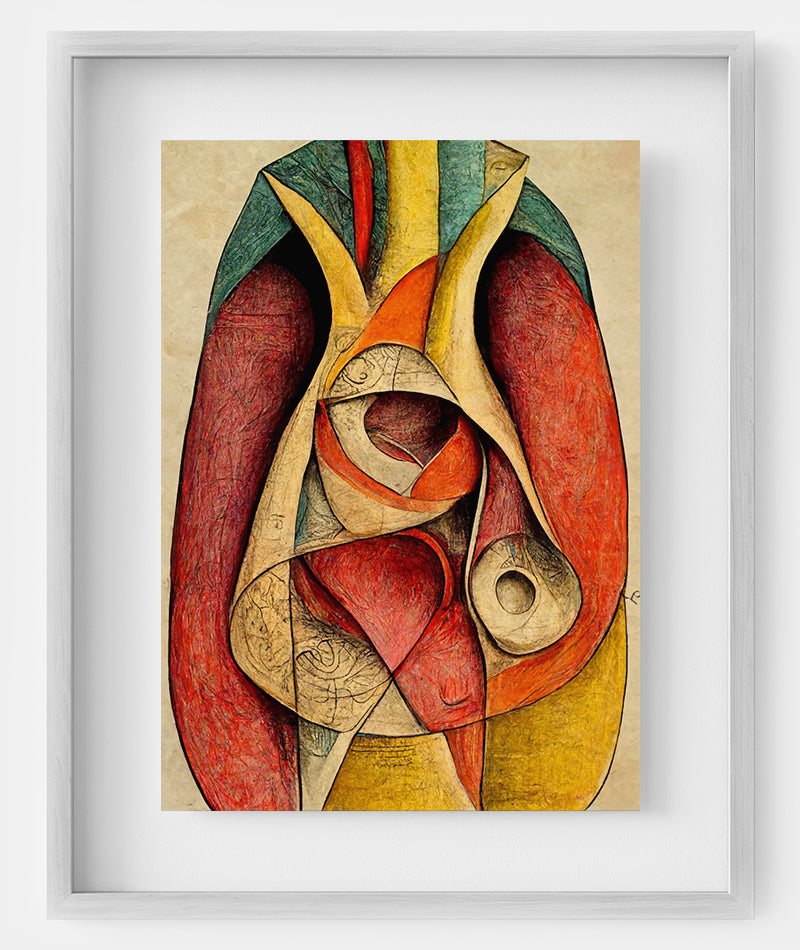The image is a vertical rectangular photograph of a modern abstract painting, enclosed in a light gray, silver-painted wooden frame, and mounted against a white wall. The artwork is surrounded by a 2-inch white matting that accentuates its vivid colors. The painting itself is an abstract expressionist piece, characterized by its bold and erratic use of multicolored shapes and lines. The background of the painting is a cream color, strikingly contrasted by an intricate mixture of paint, colored pencils, and pen. The main focal point is an oval shape with an almost anthropomorphic quality, suggestive of a face. At the top, there is a green cap-like figure, flanked by red sections curving downward on both sides. Below the red areas are gold curved shapes, leading to a central gold three-pronged figure that resembles an eye, with a red, tongue-like form hanging down. The abstract arrangement and vivid colors invite viewers to see various recognizable forms, such as a human heart, a chicken face, or even a tomato plant, making it a rich and engaging piece to ponder.